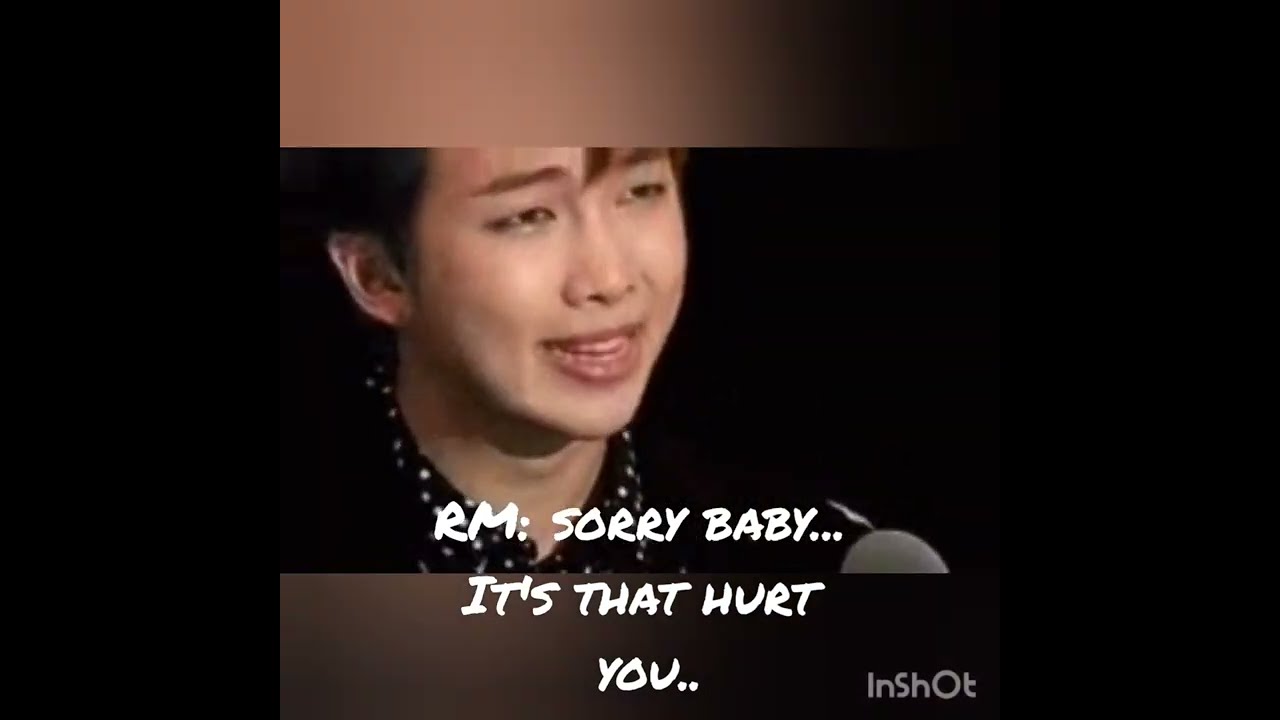The photograph depicts an Asian man with a light complexion, teary eyes, and slightly squinted brown eyes, staring forward and a bit to the right. His mouth is partially open, revealing both the top and bottom rows of teeth. The man's black hair partially covers his left ear, with bangs falling between slightly raised eyebrows. He wears a black collared shirt adorned with white polka dots, and possibly a black blazer. In front of him, towards the lower right, is the edge of a microphone. Text overlays the image, reading "RM: sorry baby... it's that hurt you.." in white letters. The bottom right corner contains the logo "in shot" in gray letters. The image is framed with solid black strips on the left and right, and blurry strips at the top and bottom, creating a high-definition TV shape. The entire background is black, enhancing the focal point on the man's emotional expression.